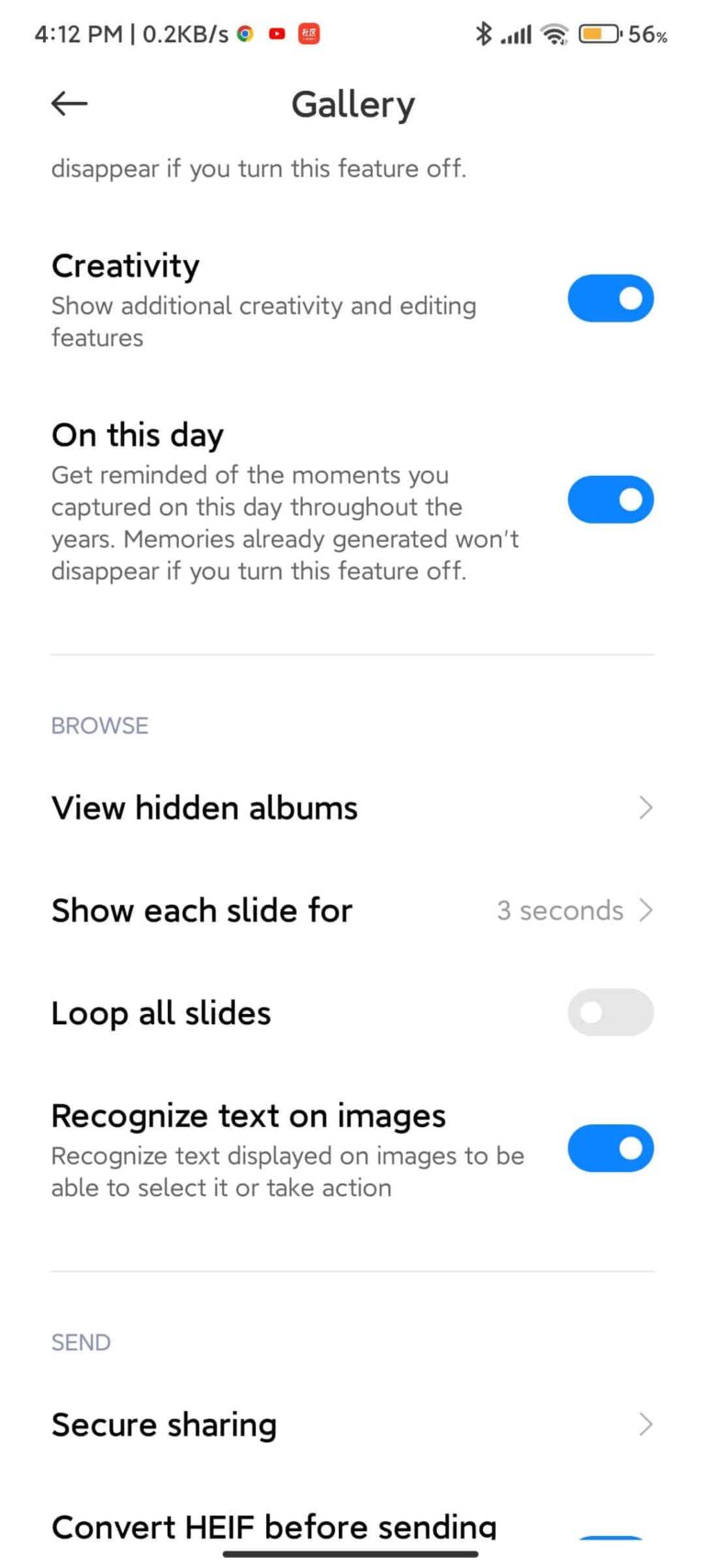This image portrays a detailed screenshot of a gallery application interface taken on October 12, at 4:12 PM. The file size is 0.2 KB and the device's battery is at 56%, with a stable connection indicated.

The top portion of the image displays the gallery, with options to manage display features and editing tools. A message under the gallery section informs users that their memories will persist even if some features are turned off. The creativity enhancement features, including additional creative editing options, are enabled. The 'On This Day' feature allows users to be reminded of moments captured on the same date in previous years.

In the browsing section, options include viewing hidden albums and setting slideshows to show each slide for 3 seconds. However, the "Loop all slides" feature is currently turned off. The application also has a built-in text recognition feature, allowing for text within images to be selected or actions to be taken, and this feature is enabled.

The sending options incorporate secure sharing, with an arrow indicating further options. There's also an option to convert HEIF format images before sending, which is indicated with a blue line but lacks additional icons or circles.

Overall, all the necessary features are activated, ensuring a comprehensive and user-friendly gallery experience.